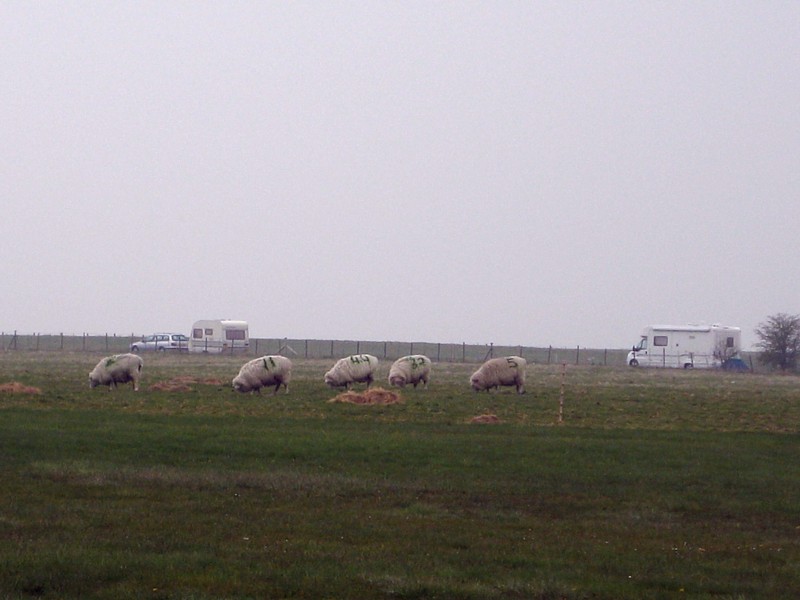In this photograph, taken on a very overcast or foggy day with a light gray sky, a group of five fuzzy sheep graze in a green field scattered with yellow hay. Each sheep has a dark green or black number painted on its side, including 11, 44, 32, and 5, with one unclear. All the sheep are facing left with their heads down, eating the grass. In the background, there is a medium-sized, two-axle RV near a tree on the right, and a small, towable camper attached to a silver or white station wagon. The field is bordered by vertical posts of a barbed wire fence.